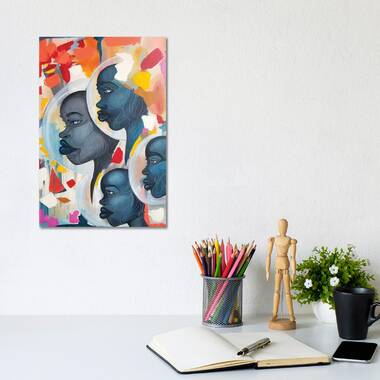The image portrays an artistic workspace meticulously arranged on a light-colored countertop or desktop, set against a pale gray wall. In the bottom section of the image, an open white notebook with a black binding sits prominently on the surface, accompanied by a silver metal pen resting on it. To the right of the notebook lies a black-screened cell phone, positioned at a slight angle. Nearby, a sleek black coffee mug is placed just in front of a small white potted plant, which boasts a few delicate white flowers amidst its green foliage. Adjacent to the plant stands a 10-inch tall wooden artist's mannequin on a circular wooden platform, ready to aid in anatomical studies. Further to the left, a mesh jar overflows with a vibrant assortment of colored pencils.

Dominating the top left corner of the image is a modern painting featuring four dynamic profiles of women's faces, all gazing leftward. The artwork is rich in color, with splashes of red, blue, yellow, purple, and white creating an engaging and lively backdrop. The overall scene is very clean and suggests an organized and inspirational creative space.